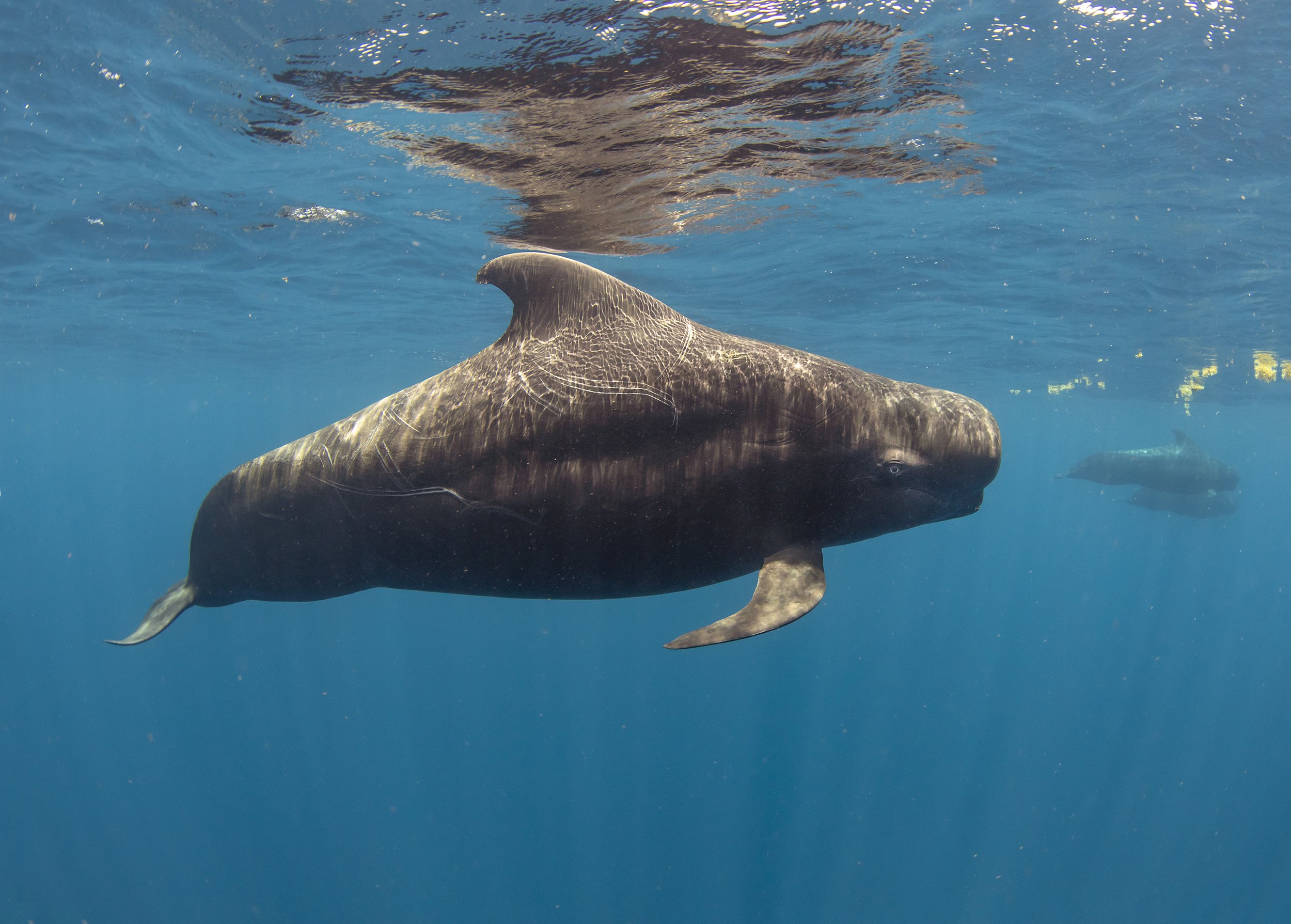This detailed, full-color, square photograph captures an underwater scene bathed in natural daylight, framed by the clear, blue expanse of the ocean. Near the water's surface, where ripples create a shimmering effect, a prominent small whale is the focal point of the image. The whale, identified as a pilot whale, features a distinctive curved dorsal fin akin to that of a dolphin or shark, and its stubby body is marked with white lines that may resemble scars. The whale is swimming towards the right, and its reflection can be seen on the water’s surface, creating a grayish mirror image. In the background, towards the center and right middle of the image, two more pilot whales can be seen, accompanied by faint bubbles and striations in the water. The ocean's clarity highlights vertical rays and shades of blue that give depth to this captivating marine scene.